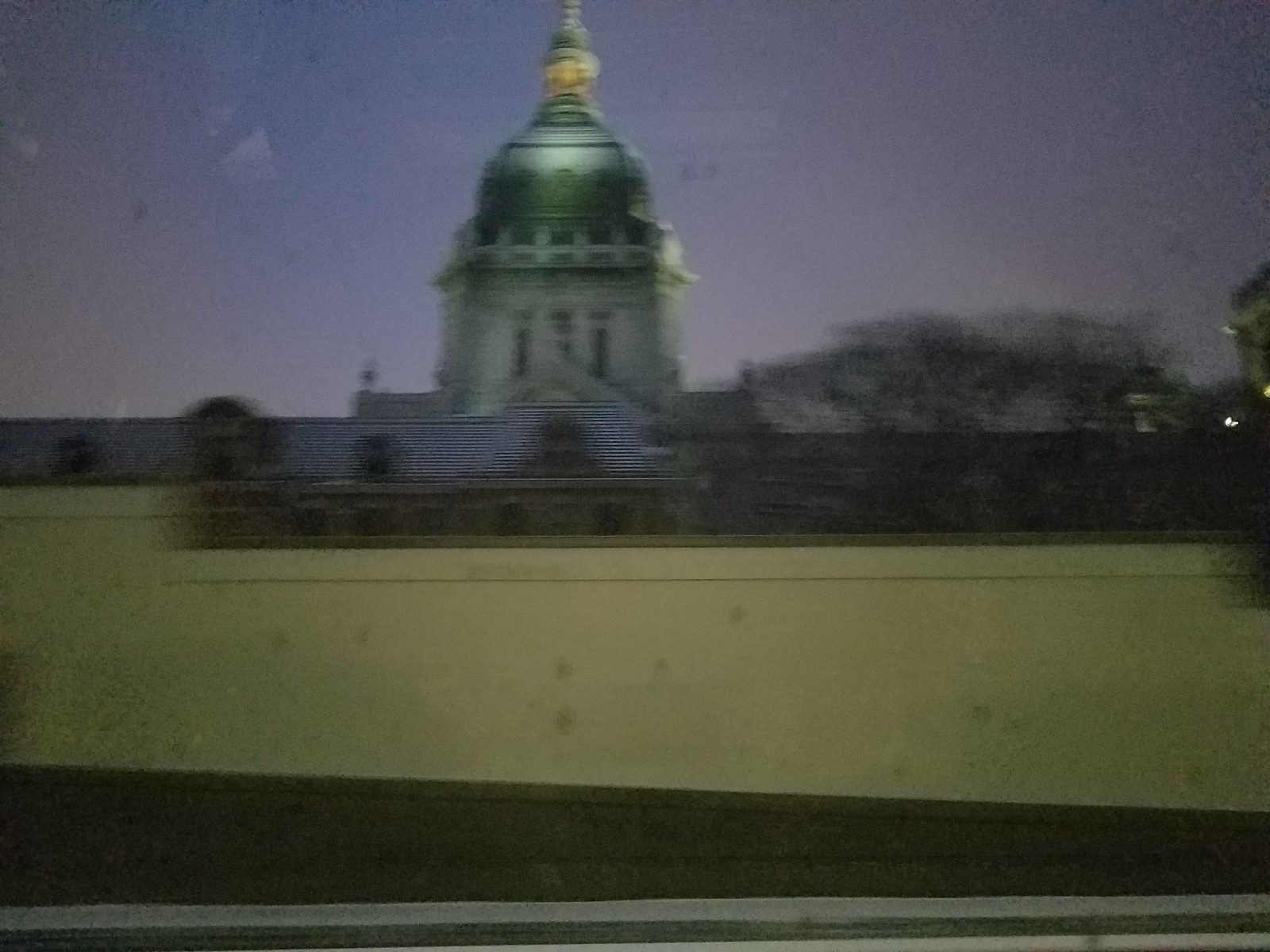A slightly blurred photograph captures a majestic domed building positioned towards the center top of the image. The building, primarily of grayish-white color, features a prominent green dome accompanied by a smaller beige dome, characterized by a yellowish hue. Atop the structure, a spire is visible, though its peak extends beyond the frame. The facade hosts a series of elongated rectangular windows, though details below these elements are indiscernible due to the blurring. In the foreground, a light green wall-like structure runs horizontally across the image, transitioning to a darker green below. To the right, blurred foliage suggests the presence of trees.